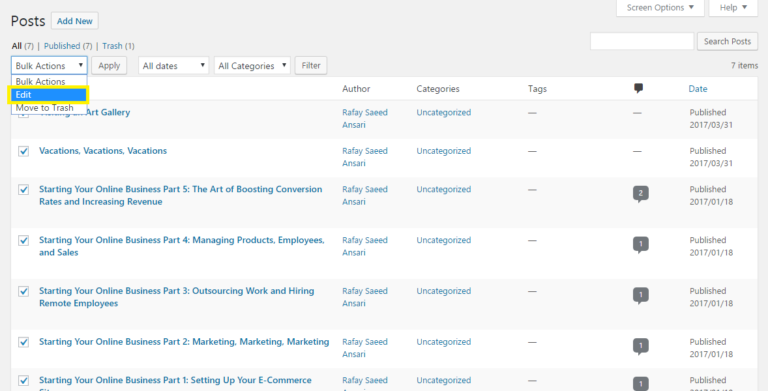The image features a gray background with a zoomed-in and slightly blurry view of a user interface, making the elements difficult to see. In the top left corner, the word "Post" appears in black text, accompanied by a button. Below it, blue text reads "Add New," followed by options indicating "All (7)," "Published (7)," and "Trash (1)." On the top right, two drop-down menus are visible: one labeled "Screen Options" and the other labeled "Help." Beneath these, there's a white box with a "Search Posts" button next to it.

Positioned on the left side, under the "All" section, another drop-down menu appears, labeled "Bulk Actions." This menu has options such as "Edit" and "Move to Trash," with "Edit" highlighted in blue and surrounded by a gold border. Adjacent to the bulk actions menu is an "Apply" button. Further to the right, another drop-down menu labeled "All Dates" is present, followed by an "All Categories" menu, and finally a "Filter" button.

Below these menus, various columns are displayed: "Author," "Category," "Tags," and "Date," providing organizational details for the posts.